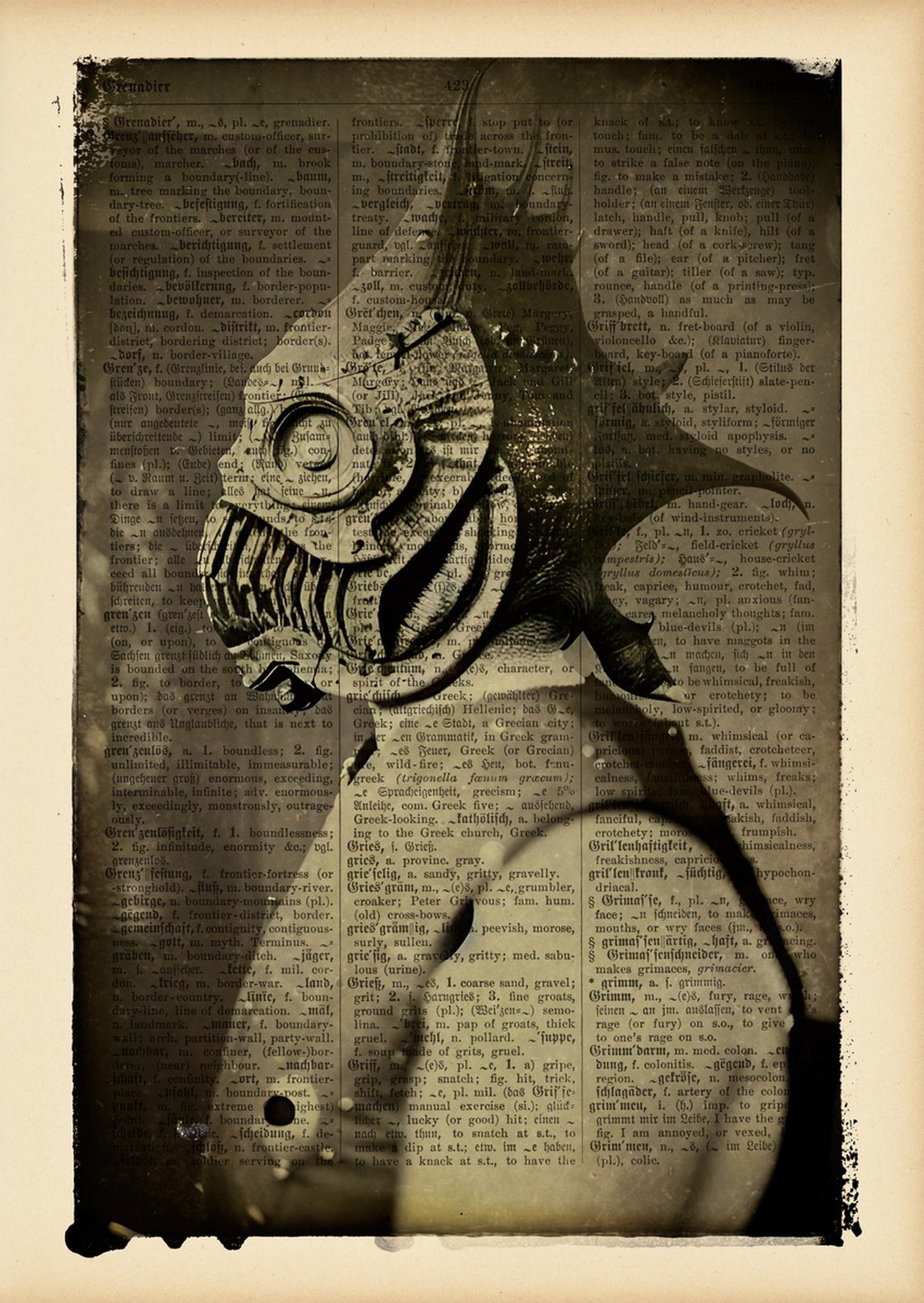This artwork features a sepia-toned, steampunk-inspired portrait set against a background that resembles aged, faded dictionary or encyclopedia pages. The central figure is a man shown in side profile, dressed in a white collared shirt beneath a sleeveless vest. The man's head is encased in an intricate, unsettling helmet that is designed to resemble a demon-like fish or piranha. This helmet has sharp, spiky teeth, round eyes, gill-like structures on the sides, and a pointed rear mimicking a fish tail. The entire composition is bordered with a cream edge, enhancing its vintage aesthetic. The overlay of text columns adds an additional layer of complexity and depth to the artwork, making it both eerie and engaging.